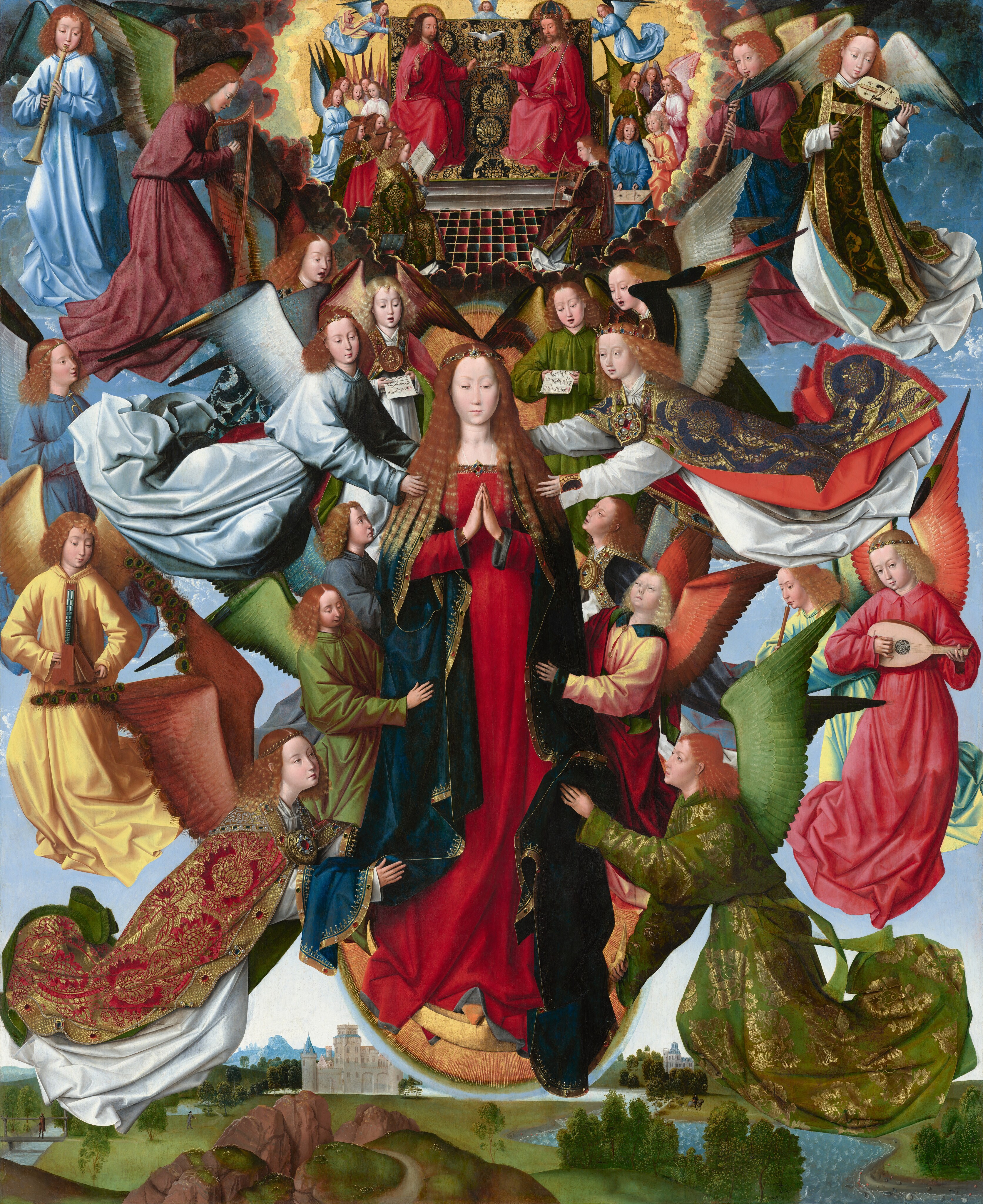The image is a richly detailed, vibrant portrayal, likely either a painting or a digital creation rather than a photograph. At the center of the composition is a Caucasian woman with long brown hair, parted down the middle, wearing a striking red dress and a heavy blue coat. She stands out with her hands clasped together in a gesture of prayer and her eyes closed, exuding a serene, spiritual demeanor as she floats in a bright blue sky above a lush green landscape featuring a tall building and trees.

Surrounding the central figure are numerous angelic and saintly individuals, all with wings and dressed in an array of colorful robes ranging from red, green, and blue to gold and yellow. These figures include both men and women with long hair, exuding a divine and ethereal quality as they float through the air. Many of these figures are engaged in playing musical instruments; on the right, a woman plays a guitar, while others play violins, flutes, and brass instruments such as trumpets both in the upper corners of the image.

Above the central woman, perched on an altar or throne-like structure, sit two men in red robes. They are flanked by blue angels and are connected by a dove flying between their hands. Additionally, various women on either side of the central figure are depicted in positions of musical and spiritual engagement, enhancing the celestial and harmonious atmosphere of the scene. The overall composition is clear and luminously detailed, with the bright blue sky and white clouds providing a transcendent backdrop for this divine assembly.